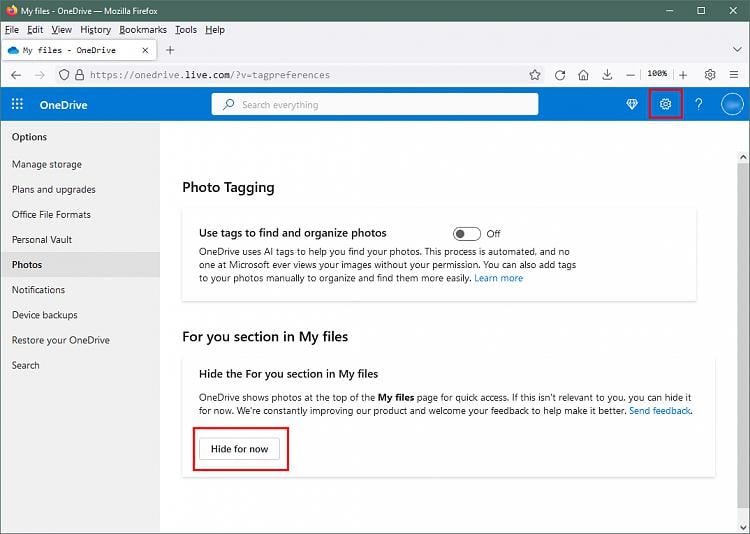A person is viewing their OneDrive account on a Firefox browser. The screen shows "My Files - OneDrive - Mozilla Firefox" in the upper left corner on a medium grey background. The browser's menu bar below this displays options: File, Edit, View, History, Bookmarks, Tools, and Help. 

The "My Files" section, marked by a blue cloud icon, is selected. Directly below the label, the URL bar displays the current web address, with typical browser icons like Download, Home, Refresh, and Bookmark Star visible. 

The header of OneDrive features a blue background containing a search field labeled "Search Everything," a diamond icon to the right, and a gear icon highlighted with a red rectangle. The main section of the screen consists of various options on the left sidebar: Options, Manage Storage, Plans and Upgrades, Office File Formats, Personal Vault, and Photos (currently selected, indicated by a grey background). Additional options include Notifications, Device Backup, Restore Your OneDrive, and Search.

On the right side of the main area, the "Photo Tagging" section is visible, explaining how tags can be used to find and organize photos. The toggle next to this feature is set to the off position. 

Further down, there’s a section titled "For You" in My Files, which can be hidden. Below the section title is descriptive text and a button labeled "Hide For Now," which is also highlighted with a red rectangle.